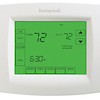The image features a compact, white, and mostly rectangular thermostat with a green digital display. Due to the small size of the image, finer details are difficult to discern, but the main elements are clear. Dominating the center-left portion of the screen is the number "72," indicating that the temperature is set to 72 degrees Fahrenheit. To the right of this primary display, another smaller "72" is visible, accompanied by up and down arrows, confirming that the current room temperature also matches the set temperature at 72 degrees Fahrenheit. Below this, the number "630" is visible, potentially indicating the time or a scheduled event, though the exact meaning remains unclear due to the image's small size. Additional text and elements are present on the display, particularly below the number "630," but they are indistinct. Overall, the white thermostat with its green digital screen is accurately managing the room temperature, maintaining it at a consistent 72 degrees.